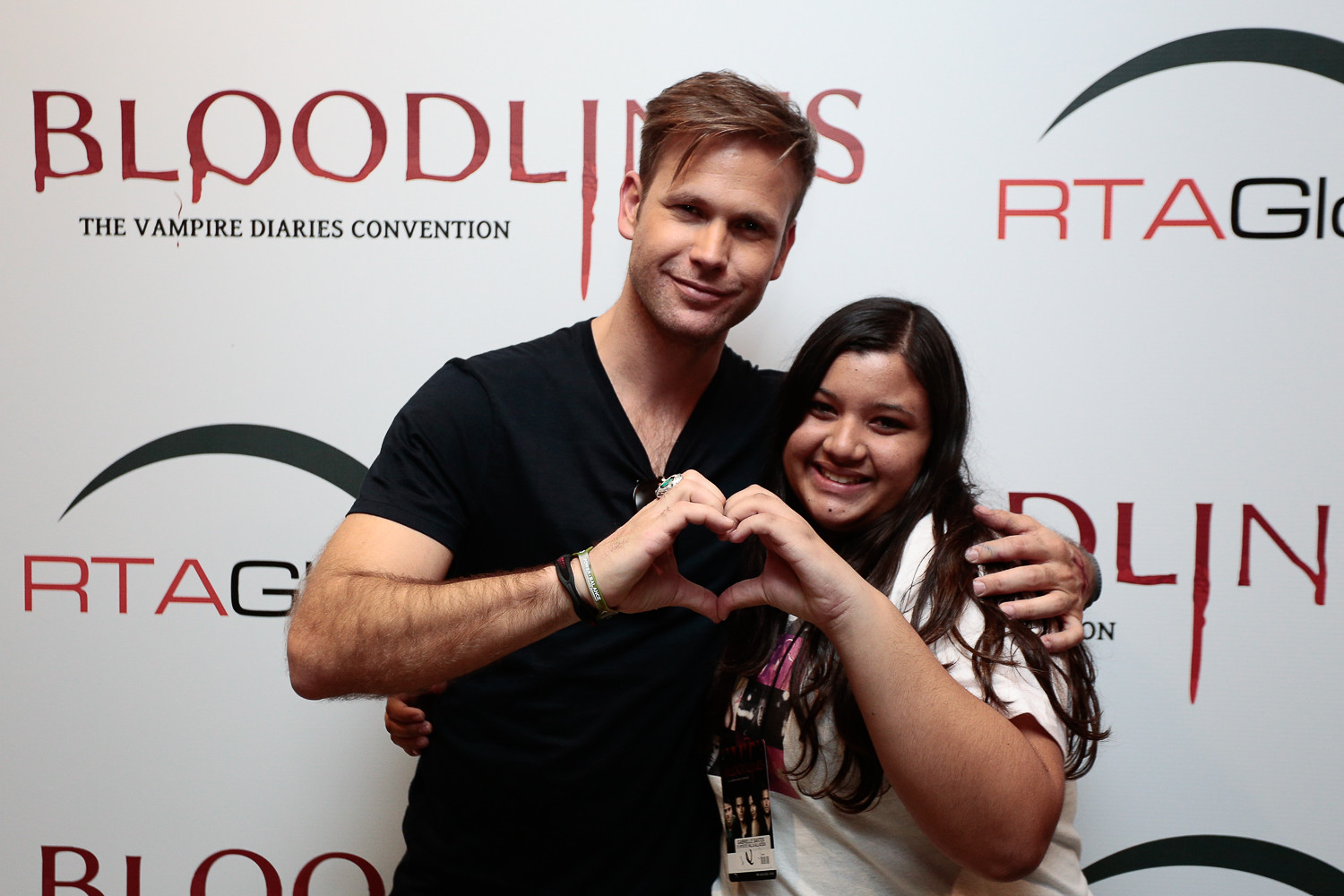In the image, two individuals are posing in front of a recurring white backdrop with text and logos in red and black. The text features "Bloodlines" in a blood-like drip font above "The Vampire Diaries Convention," with additional partially visible letters "RTA GL." A curved black line also adorns the backdrop. The pair in the foreground are making a heart shape with their hands. The person on the left, a man with short brown hair, is wearing a black v-neck short-sleeve t-shirt and has accessories that include a white and black wristband and a silver ring with a green detail. He is also placing his arm around the shoulders of the person on the right, a woman with long black hair. She is smiling broadly and is dressed in a white t-shirt with a graphic that is partially obscured by a lanyard hanging around her neck. Both appear cheerful, contributing to the warm atmosphere of the photograph.